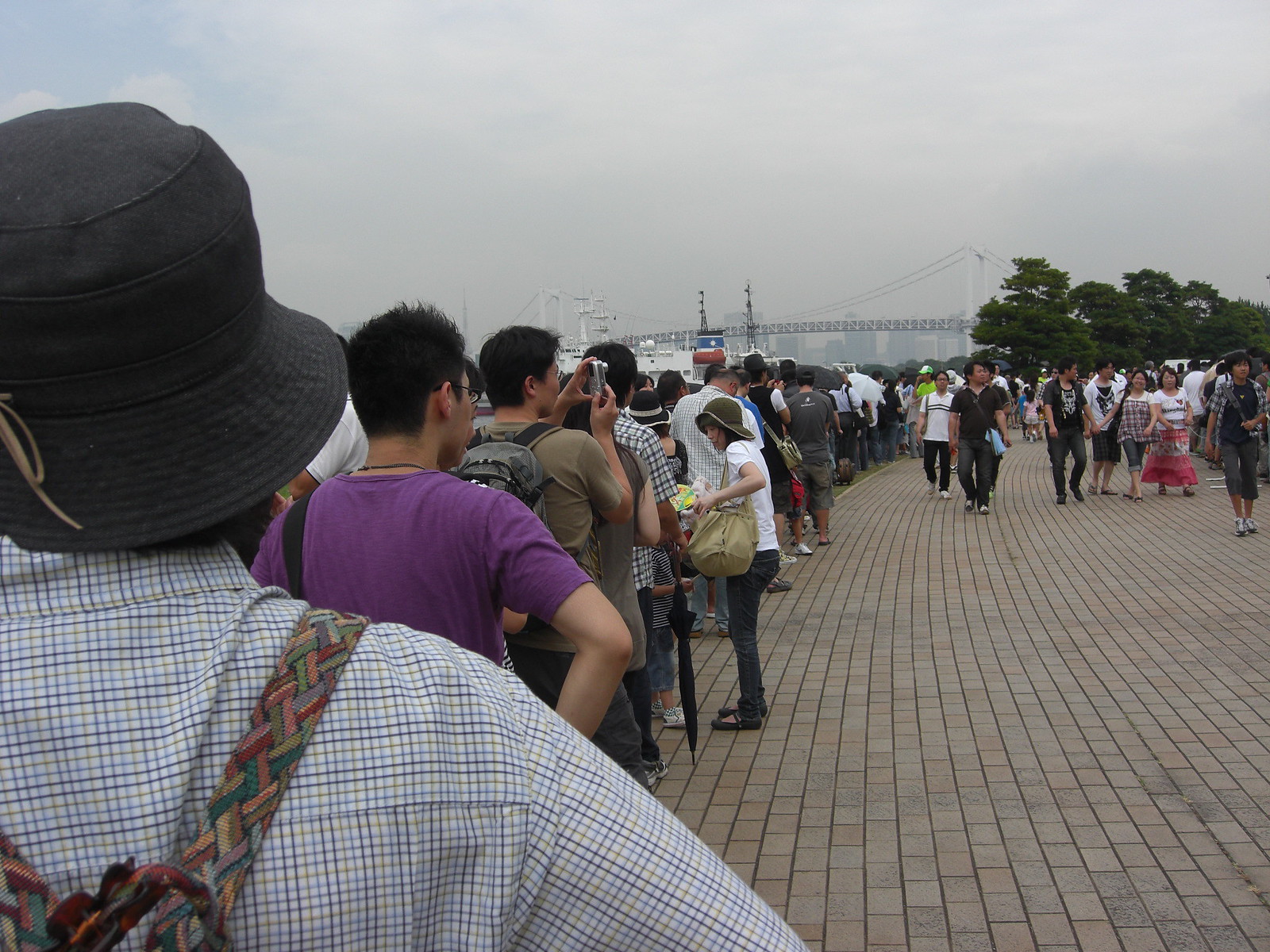This outdoor photograph captures a bustling brick walkway lined with people, likely tourists, who predominantly appear to be of Asian descent. The scene is set under a gray, overcast sky that suggests either a cloudy day or the early twilight hours. On the left side, a long queue of individuals extends into the distance, with the person closest to the camera wearing a black hat, a blue checkered shirt, and a multicolored backpack. Directly ahead of them stands someone in a purple short-sleeved shirt with short black hair and glasses. The background reveals a bridge arching over a waterway, possibly a lake or river, indicating an urban setting somewhere in Asia. The right side of the image features a few people walking towards the camera, with some trees and a further cityscape providing depth and context to this vibrant outdoor scene.